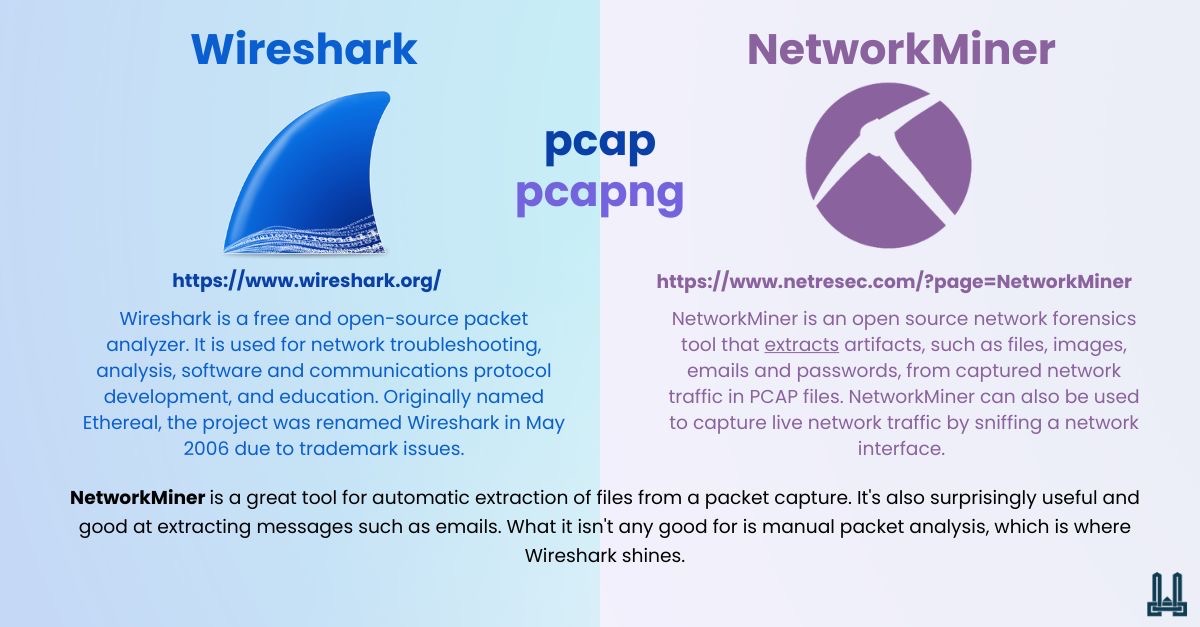The image is a horizontally oriented rectangular flyer or webpage with a divided layout. The left side features a blue background with a prominent blue shark fin at the top, labeled "Wireshark" in blue text, followed by its website URL (https://www.wireshark.org). Beneath, a detailed paragraph describes Wireshark as a free and open-source packet analyzer used for network troubleshooting, protocol development, and education. This project, originally named Ethereal, was rebranded to Wireshark in May 2006 due to trademark issues. 

The right side of the image has a pale purple background with a symbol of a miner's axe inside a purple circle, labeled "NetworkMiner" above its website URL (https://www.netresec.com). The accompanying paragraph elaborates on NetworkMiner as an open-source network forensics tool that extracts artifacts such as files, images, emails, and passwords from captured network and PCAP files. It is noted that NetworkMiner can also capture live network traffic by sniffing a network interface.

Central to the image are two lines, "PCAP" in blue and "PCAPNG" in purple. At the bottom, a unified black text bar spans across both sections, emphasizing that NetworkMiner excels at automatic extraction of files and messages like emails from packet captures, but is not suitable for manual packet analysis, a task for which Wireshark is highly effective.